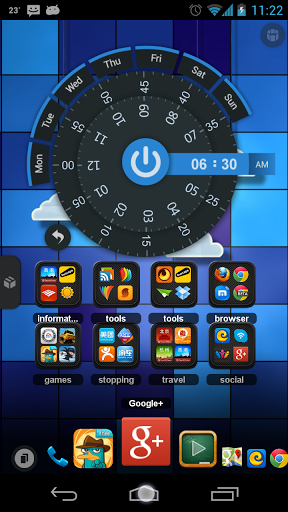The image showcases a phone screen with various icons and indicators. At the top left corner, the number "23" is displayed prominently. Moving rightward, there is a rectangular thought bubble containing a happy face. Adjacent to this, there is an image of a creature's head featuring antennas on each side. Further to the right, on the upper right corner, a gray alarm clock icon is visible, followed by a blue Wi-Fi symbol. Next to these icons is a blue bar, and to its right, a white and blue battery icon indicating the remaining battery power. The time "11:22" is displayed at the far right of the top bar. Below these elements, part of another image can be seen, though it is not fully visible in this description.